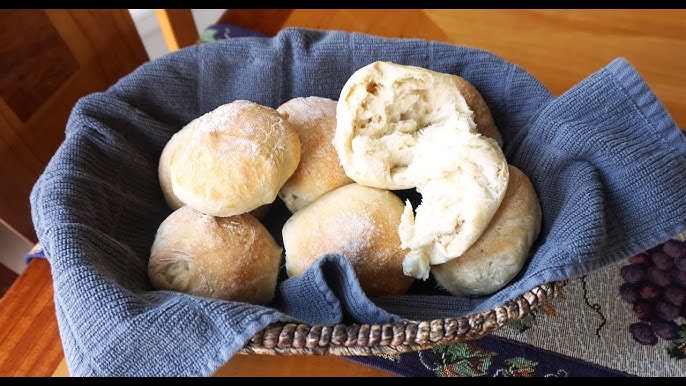This is an overhead photograph of a woven gray straw basket lined with a slate blue cloth, containing seven round and fluffy dinner rolls. The rolls, golden brown and dusted with a light sprinkle of flour, exude a warm, homey appearance reminiscent of a slight snowfall. One roll in the top right corner is torn open, revealing its soft, white interior. The basket is situated on a cherry-colored wooden table, adorned with a decorative placemat featuring a variegated gray center with bunches of purple grapes and a border with green swirly leaf designs. A wooden chair's back is partially visible on the left, adding a touch of rustic charm to the cozy scene.